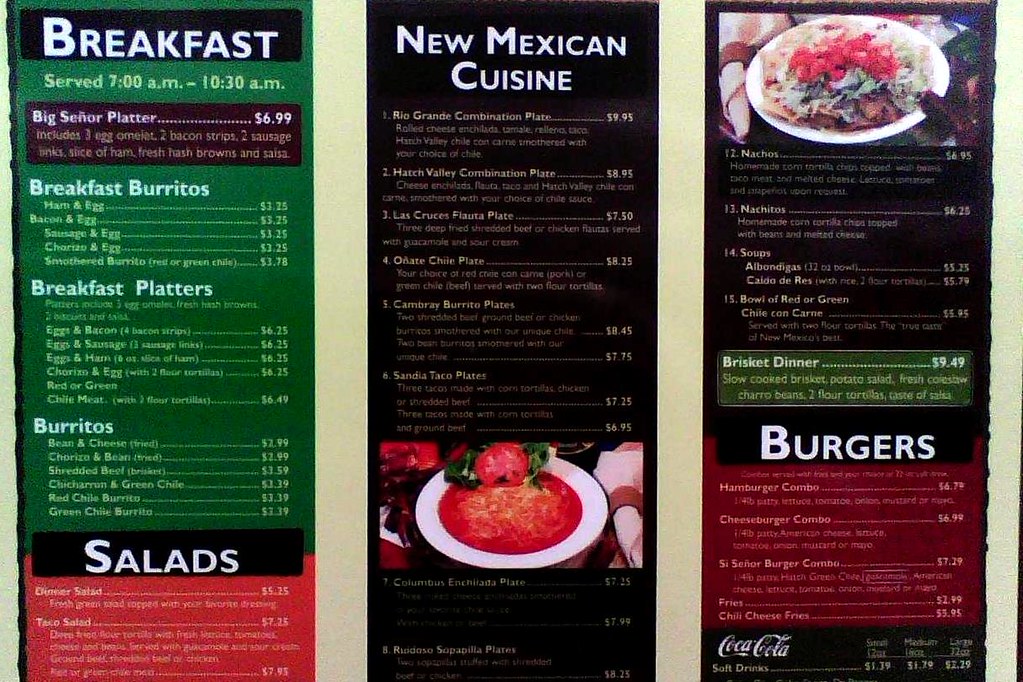In this detailed image, we observe three distinct menu sections displayed within a restaurant setting. On the left panel, the header "Breakfast" is prominently featured in white text against a black background. The primary background of this section is green, transitioning to pink at the bottom. This section lists categories such as Breakfast Burritos, Breakfast Platters, and Burritos. Below the breakfast section, the word "Salads" is also written in white text on a black background.

The central panel showcases "New Mexican Cuisine," set against an entirely black backdrop. A vividly detailed dish is visible towards the bottom, featuring a white plate adorned with red sauce, a tomato slice, and two green leaves flanking the tomato. The surroundings reflect a typical restaurant ambiance to complement the menu.

On the right-hand panel, the top portion highlights a visually appealing pasta dish, characterized by green, brown, and red tomato slices integrating at the top. Beneath this is a list of five different menu items, with the bottom item named "Brisket Dinner," displayed against a green background. Underneath the brisket item, the word "Burgers" appears in white text on a black background, followed by a red segment. The section concludes with a cut-off Coca-Cola sign, indicating the start of the drinks menu, which lists items on the left with corresponding prices on the right.